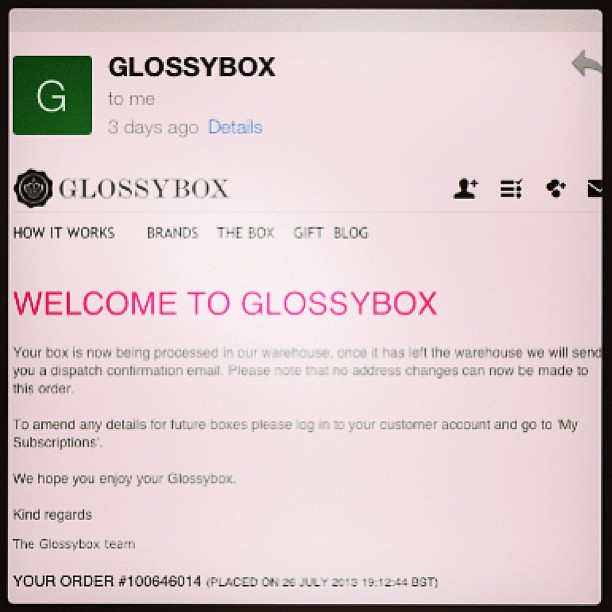The image depicts a photograph of an email displayed on a screen, evidenced by a slight glare in the middle. In the upper right corner, common email icons such as "add a person," "hamburger menu," and "reply" are visible. On the upper left, there is a green square with a white "G," next to which "Glossybox" is written, addressed "To Me" three days ago with a "Details" link in blue text. Below, a navigation menu includes sections like "How It Works," "Brands," "The Box," "Gift," and "Blog." The main body of the email begins with a pink "Welcome to Glossybox" message, followed by black text stating that the recipient's box is being processed in the warehouse and a dispatch confirmation email will be sent once it leaves the warehouse. The email emphasizes that no address changes can be made to this order, but details for future orders can be amended by logging into the customer account under "My Subscriptions." The email concludes with "We hope you enjoy your Glossybox," "Kind Regards," and "The Glossybox Team." At the bottom, the order number 100646014, placed on 26th July 2018 at 19:12:44 BST, is mentioned.